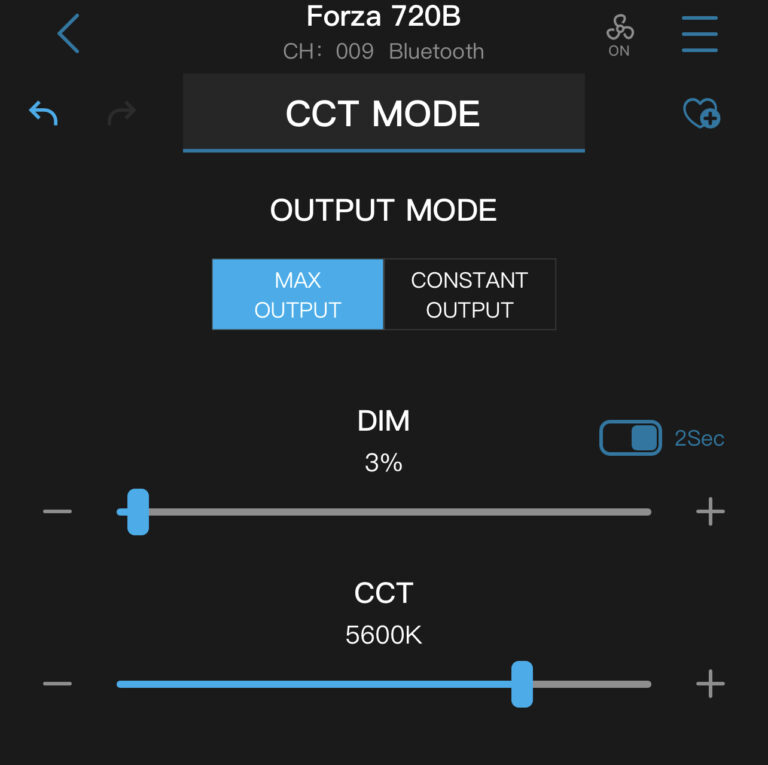### Forza 720B Interface Description

The image depicts a dark-themed interface with various controls and indicators. At the top, in bold white text, it reads "Forza 720B". Below this, in grey text, it states "CH: 009 Bluetooth".

On the left side of the interface, there is a blue arrow pointing to the left. To the right of this arrow, there is a fan icon labeled "ON" with three blue lines beneath it.

A grey box features prominently just below with the words "CCT Mode" in white text, underlined by a blue line. Further down, the interface indicates "Output Mode" in white text. This area also includes two buttons: the left button, labeled "MAX OUTPUT", is encased in a blue box, while the right button, labeled "CONSTANT OUTPUT", is encased in a black box.

The next section displays the word "DIM" in white, followed by "3%". Directly below this is a grey bar with a minus sign on the left and a plus sign on the right. A small blue marker on this bar is positioned closer to the left side.

Additionally, the interface shows the label "2 Sec" in a small box containing both dark and blue areas. Lastly, the words "CCT 5600K" are displayed, accompanied by a similar grey bar with a minus on the left and a plus on the right. This bar is mostly blue, with the marker placed closer to the plus side.